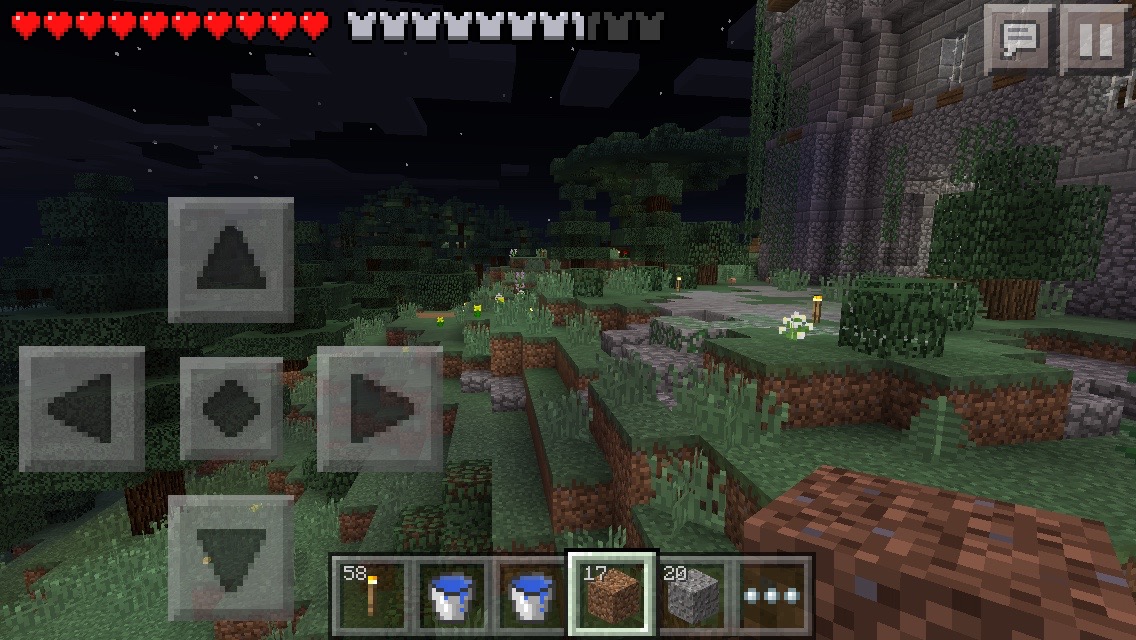This detailed nighttime screenshot of Minecraft, specifically the PocketMinecraft mobile version, depicts a player editing their in-game castle project. The image reflects the distinctive pixelated aesthetic of the game, with visible features including pixelated grass, flowers, and shrubs that form part of a garden in front of a partially completed castle. Garden steps and bricks are also visible, adding to the nighttime scene illuminated by a starry sky. The user interface clearly identifies it as the mobile version: large on-screen directional arrows are displayed on the left for movement, characteristic of touch controls, along with a centered inventory bar at the bottom showing various items such as a torch, bricks, and other materials. In the upper right corner, the usual Minecraft interface elements like the pause and chat buttons are illuminated, along with a health bar represented by red hearts and a secondary bar depicting castle towers, where the last two and a half towers are unfilled. This all emphasizes the ongoing construction and creative process within the game.